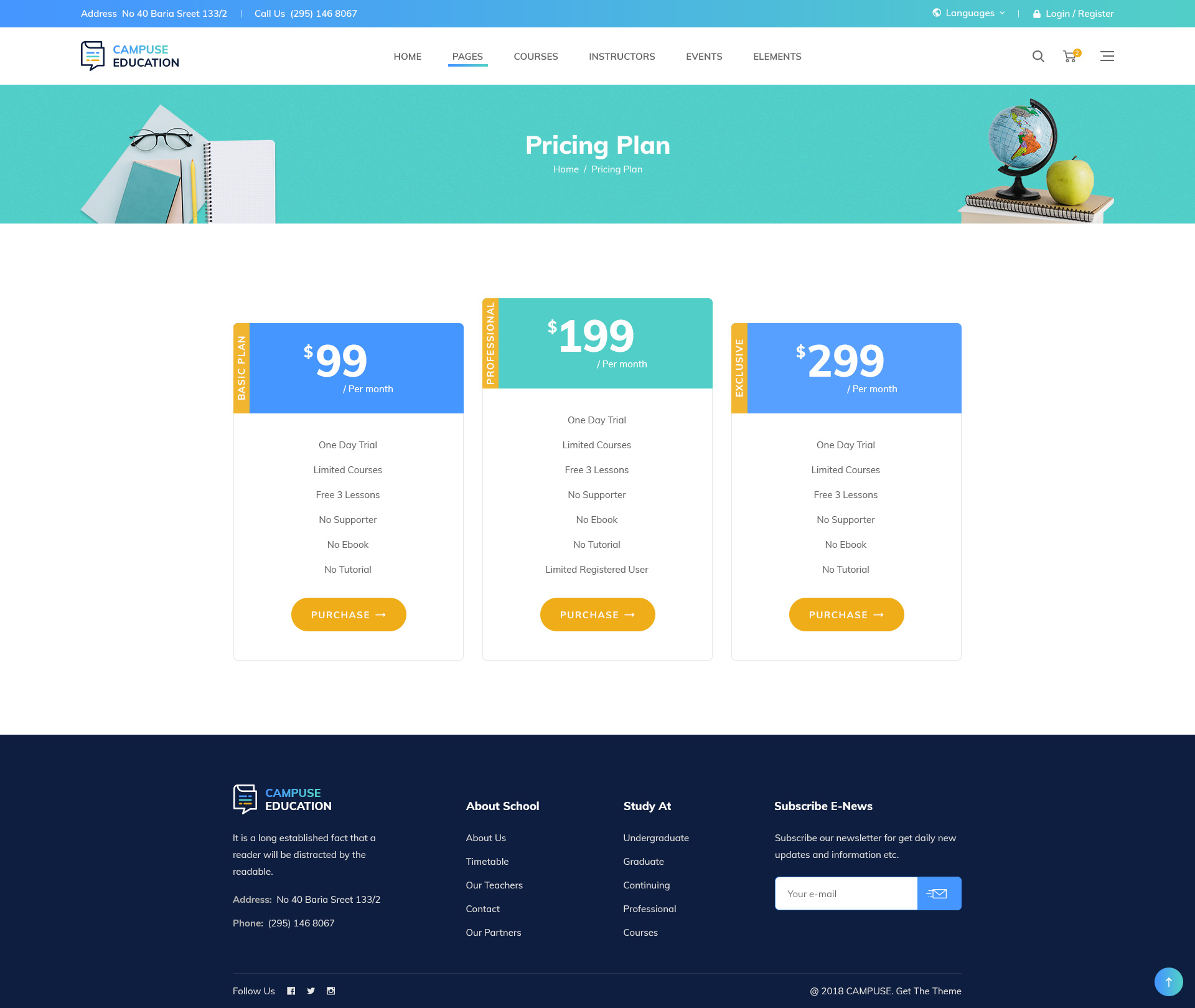The screenshot is from the website "Campus Education." The address is prominently displayed at the top in a blue stripe with the text: "Address: 40 Berea Street, 133/2." Alongside, there's a contact number: "Call Us at: 295-146-8067."

The navigation bar features six tabs: Home, Pages, Courses, Instructors, Events, and Elements, with "Pages" underlined in green, indicating the current section. Below this, a visually appealing teal banner spans across with imagery—on the left side, there are notebooks and glasses, while on the right, a globe and an apple rest atop a stack of notebooks. Centered on the banner, in white text, it reads: "Pricing Plan. Home / Pricing Plan."

Displayed beneath the banner are three distinct pricing plans in three separate boxes:
1. **Basic Plan**: The first box has a blue header and is priced at $99 per month. 
2. **Professional Plan**: The second box features a teal header and is priced at $199 per month.
3. **Exclusive Plan**: The third box has a light blue header and is priced at $299 per month.

Each plan box includes specific details:
- The Basic Plan offers a one-day trial, limited course access, three free lessons, but lacks support, an ebook, and tutorials. 
- The Professional Plan's specifics were not detailed in the voice caption but can be assumed to include enhanced features compared to the Basic Plan.
- The Exclusive Plan covers most features except it does not include support, an ebook, or tutorials.

Each pricing box concludes with an orange "Purchase" button at the bottom.